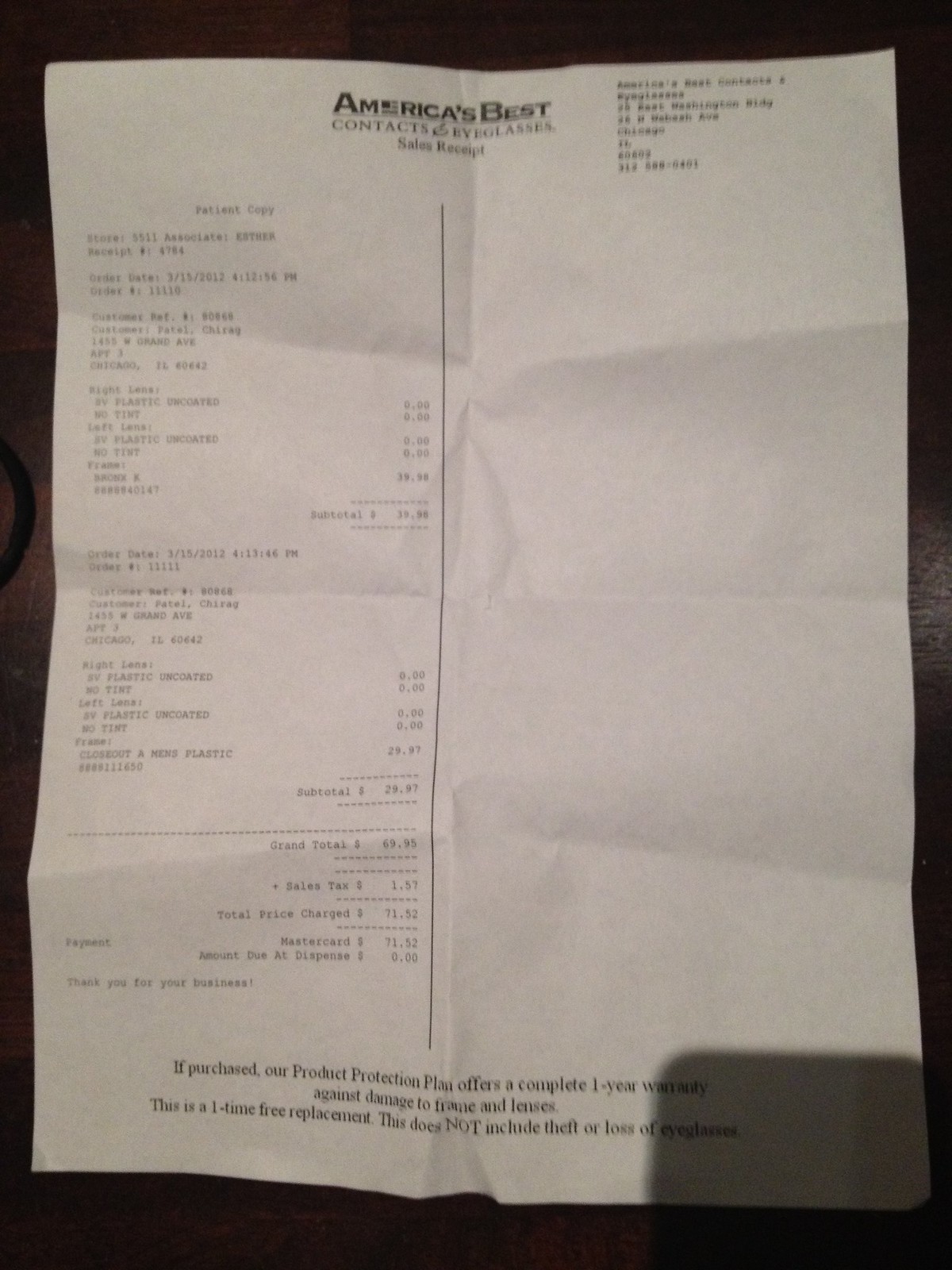This image depicts a blurry receipt from America's Best Contacts and Eyeglasses, set against a black background. The receipt is printed on white paper. At the top, it clearly states "America's Best Contacts and Eyeglasses Sales Receipt." In the top right corner, there is some illegible writing. A vertical line runs down the middle of the receipt, separating content. On the left side of this line, it is labeled "patient copy," but the rest of the text is difficult to decipher. However, detailed descriptions of services and items purchased can be perceived. To the right, financial details are listed, including a subtotal appearing to be around $29.90, sales tax, and a total charge of approximately $71 and some additional cents.